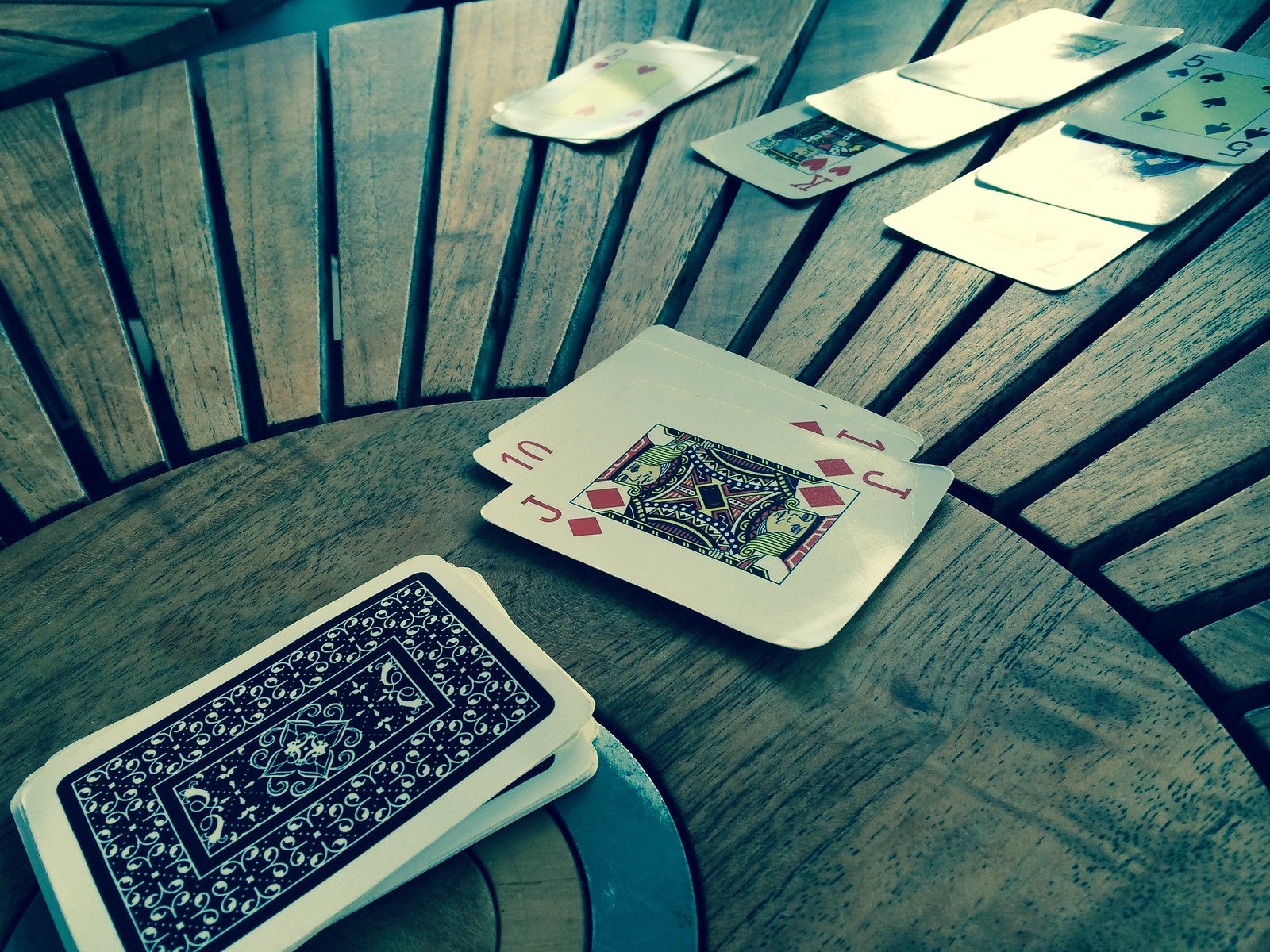The photograph showcases a uniquely designed round table with a sunburst pattern emanating from its center. The table, crafted from wood, features intricate inlays, possibly made of tiles, at its very center. Displayed prominently in the middle of the table is a stack of face-down cards, accompanied by a smaller pile of face-up cards beside it. The visible cards in this smaller stack include a Jack of Diamonds atop a Ten of Diamonds, with other cards obscured beneath. Towards the far end of the table, there are two additional rows of three cards each, partially illuminated by a light source from the top right. Despite the glare, a Five of Spades and a King of Hearts are discernible. To the left of these rows lies a tiny stack of two cards, the top one being a Two of Hearts. The entire scene is bathed in a bluish-green tint, adding a slightly ethereal quality to the image.